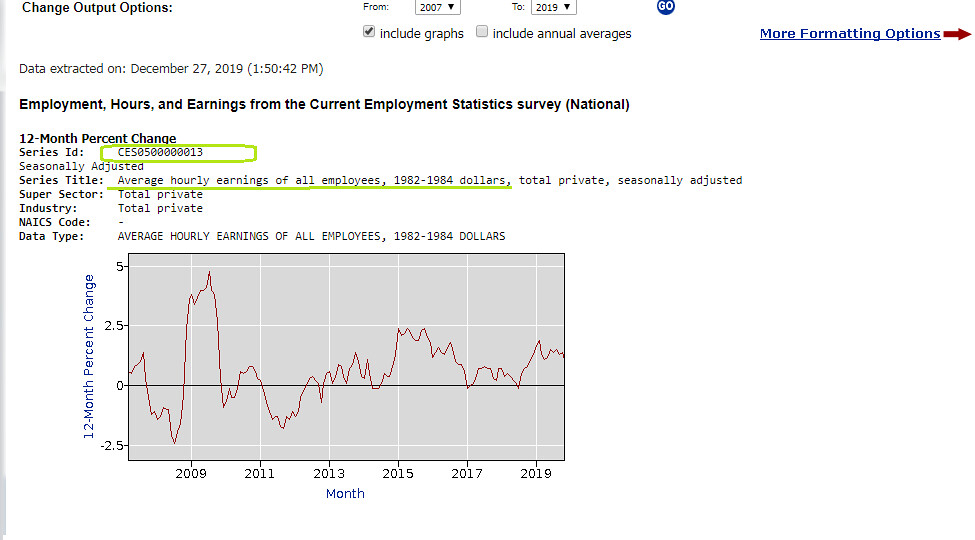The image depicts a detailed chart from the Current Employment Statistics Survey National, focusing on employment hours and earnings data. The time range is set from 2007 to 2019, with options to include graphs checked and annual averages unchecked. There is a link titled "More Formatting Options" in blue font, indicating additional settings. The data was extracted on December 27, 2019, at 1:50:42 PM.

The chart shows the 12-month percent change in average hourly earnings of all employees, seasonally adjusted, measured in 1982-1984 dollars, for the total private industry sector. The series ID is CES0500000013, and the vertical axis of the graph ranges from -2.5% to 5% change. Along the bottom, the horizontal axis lists the years from 2009 to 2019.

A red line representing the 12-month percent change fluctuates prominently, with peaks reaching up to 5% and troughs dropping to around -2.5%, notably around 2008-2009. The graph illustrates the volatility in employment statistics over the selected years.